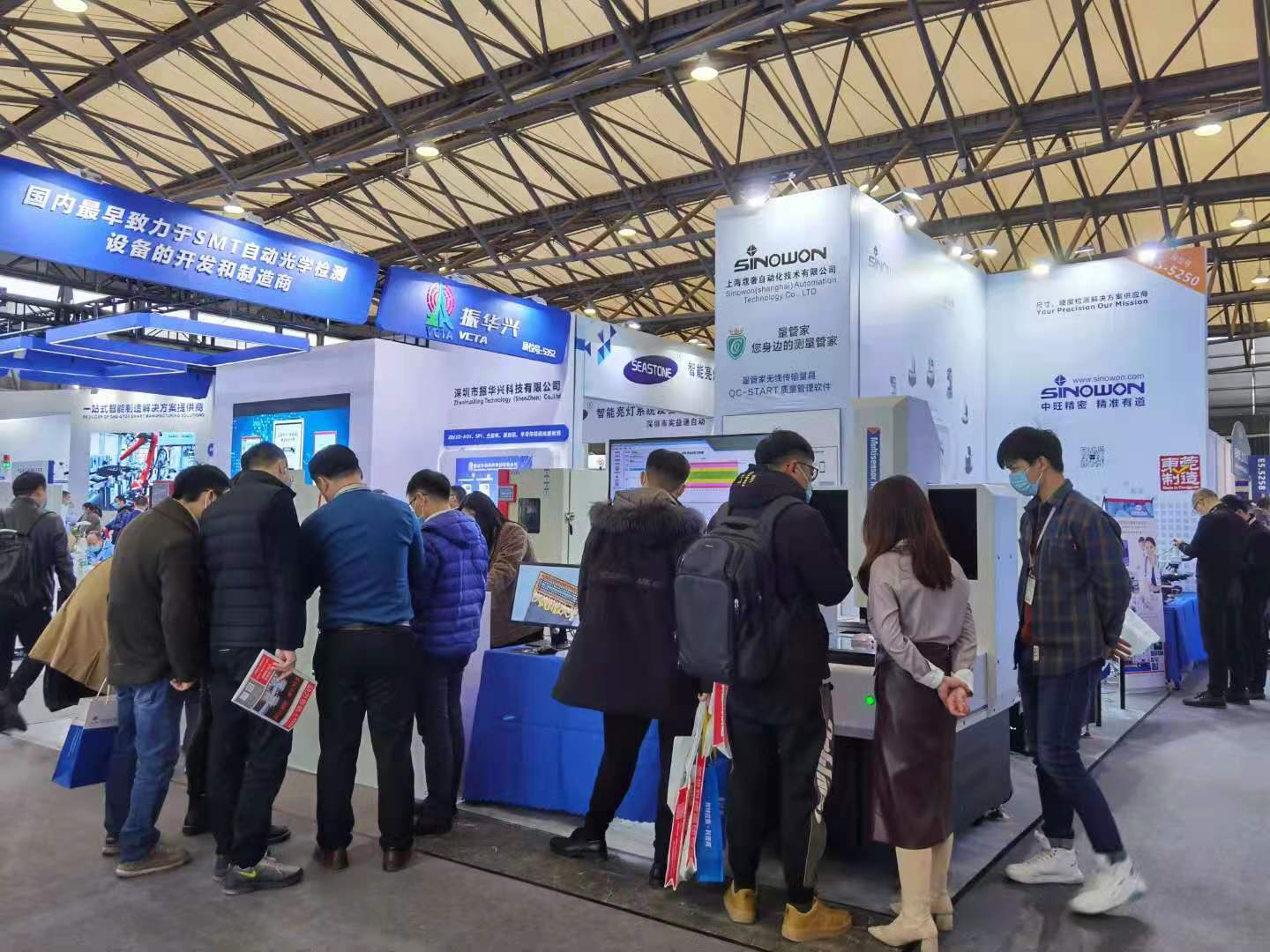The color photograph captures a bustling trade show or convention set in a spacious warehouse-like building. The venue features numerous temporary sales booths, predominantly white with blue text and banners, showcasing brands and products, with one notable brand, SINOWON, displayed in Roman letters amidst primarily Chinese and Japanese characters. The ceiling reveals rafters with light brown glass panes and hanging lights, illuminating the event space.

In the center of the image, two distinct groups stand in front of separate kiosks. On the left, five people, all of Asian descent, are positioned before a booth with a white wall, a monitor, and Japanese writing. Among them, a man in a dark blue coat stands beside another in a black puff coat holding a red and white brochure. Adjacent to them, a man in a blue sweater stands near another individual holding a blue shopping bag.

To the right, four participants gather at another kiosk facing a machine encased in white. A woman in a long skirt and long-sleeve shirt with tan boots is visible from behind, alongside a man in sneakers and a face mask. They are accompanied by a man carrying several bags, donning a black backpack and glasses, his face turned away from the camera, and another man in a black coat.

Surrounding the main groups, additional attendees mill about, reinforcing the busy atmosphere typical of such events. The overall scene is vibrant and dynamic, underscored by the various displays and the diverse, yet uniformly Asian, crowd.